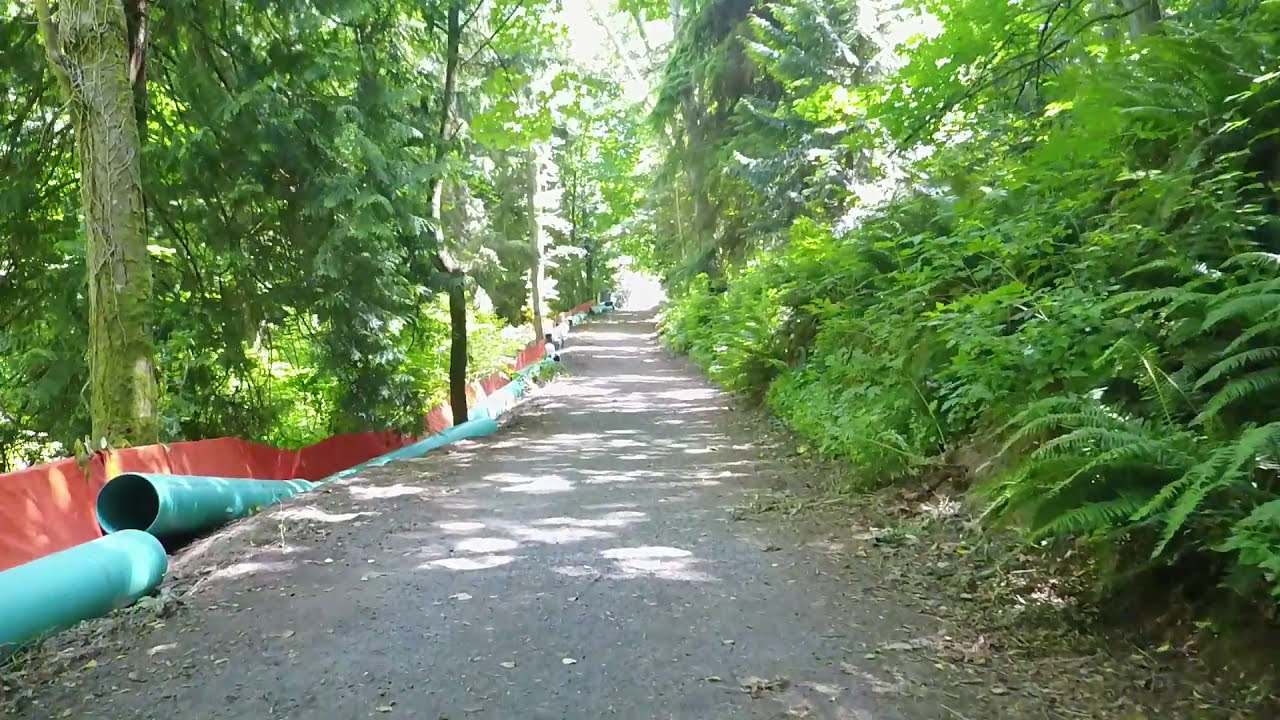The image depicts a serene, slightly uphill gravel path that winds through a lush, green landscape. On the left side of the path, there's evidence of construction work, with green sections of pipe lying around, likely to be buried underground. Leaning on the left side is an orange or red concrete wall, adding a stark visual contrast against the greenery. This wall appears to separate the path from the adjacent trees. The path itself is strewn with leaves, debris, sticks, and rocks in the foreground. There is an untrimmed, overgrown area of plants and trees flanking the right side of the path, contributing to the natural, untouched feel of the scene. The sun is shining, with its light creating reflections along the path and filtering through the branches. Notably, the scene is devoid of people or animals, emphasizing the quiet, untouched nature of this landscape.